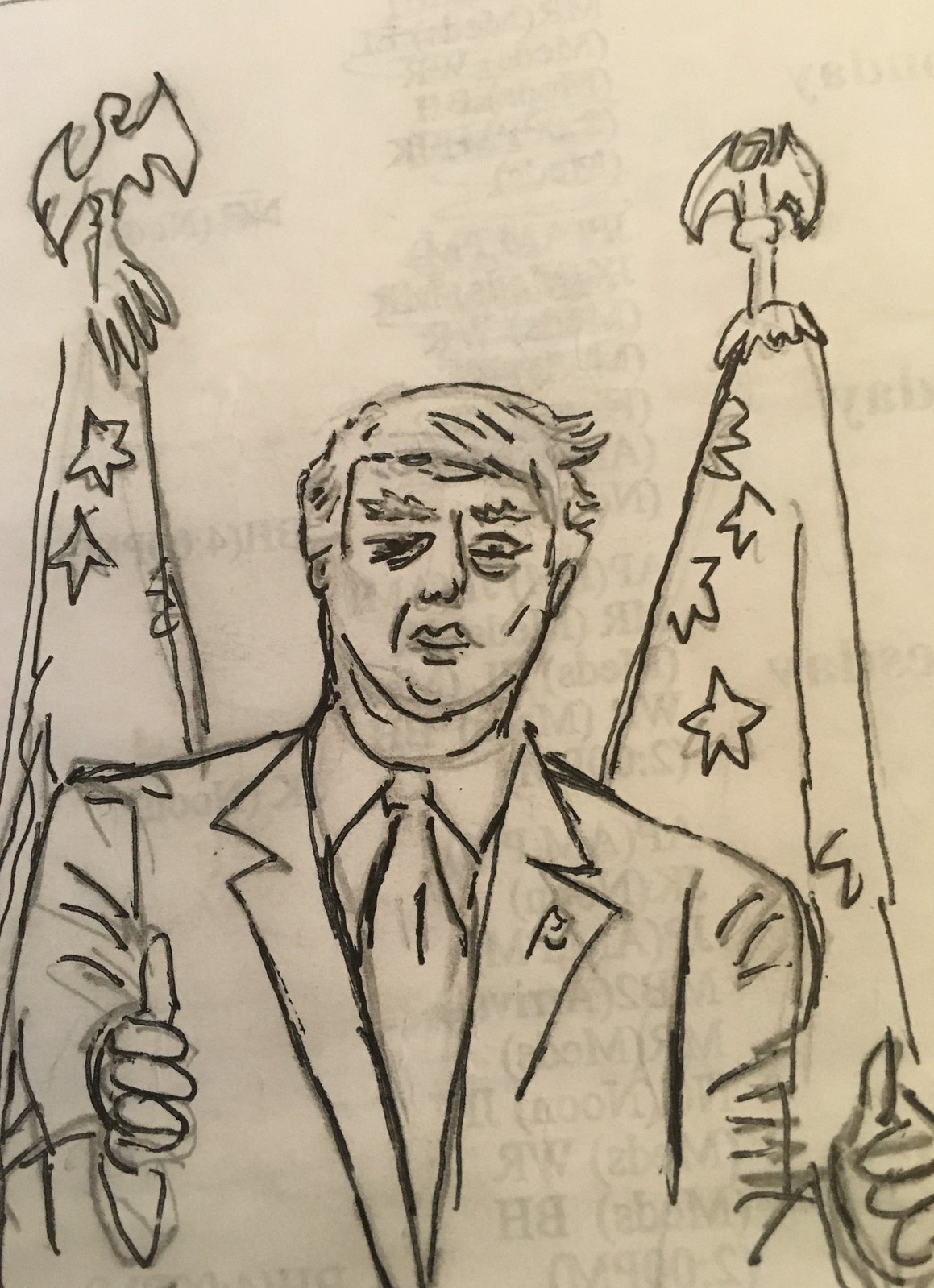This is a hand-drawn style image of a presidential-looking figure, likely a facsimile of Donald Trump, depicted on a dusty rose-colored paper using either charcoal or pencil. The figure, with unkept iconic hair and large bushy eyebrows, dons a blazer with a flag pin on the left lapel, a dress undershirt, and a wide tie. The character stands with both thumbs up, one eye partially closed in a neutral or slightly expressive facial countenance, showing finely drawn wrinkles etched into his face and jacket. In the backdrop, there are sketches of U.S. flags adorned with stars and topped with ornamental eagles. Additionally, there is a faint outline of a dress with a frilly white collar on a coat rack and some illegible writing visible through the paper, giving a faint impression of being on a schoolbook or similar context.